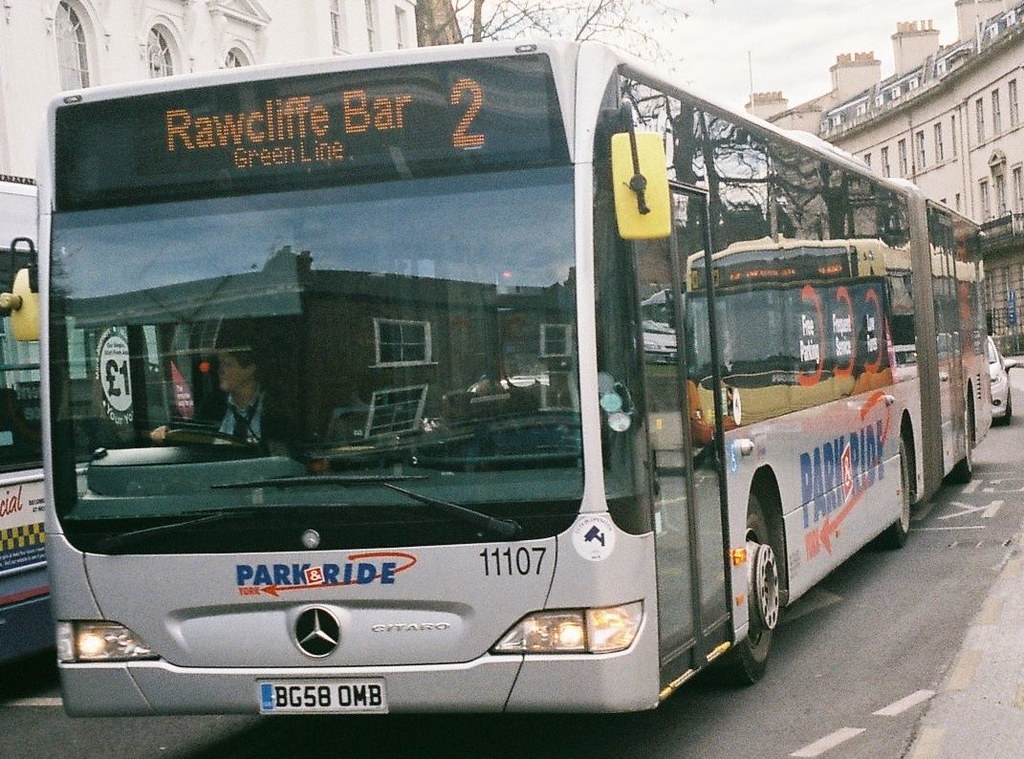The image captures a bustling city street dominated by a silver city bus prominently in the foreground. The bus, a Mercedes model, displays "Park Ride" in blue text along with an orange, curved arrow emblem on both the front and side. The digital display on the top reads "Rock Cliff Bar 2, Green Line." The license plate, BG58OMB, is visible below the Park Ride emblem, and the bus bears the fleet number 11107. Its headlights are on, and the driver's figure is discernible through the front windshield. Reflective surfaces on the bus show glimpses of another bus to its right side and a partial view of a different bus on its left. The street is marked with white lines on a gray road surface. In the background, several white buildings with brown-tiled roofs and chimney-like stacks are visible, along with their distinctive curved archway windows, indicating both residential and business purposes. A white car is positioned behind the bus, and tall, white buildings frame the scene on both the left and right upper corners of the image.